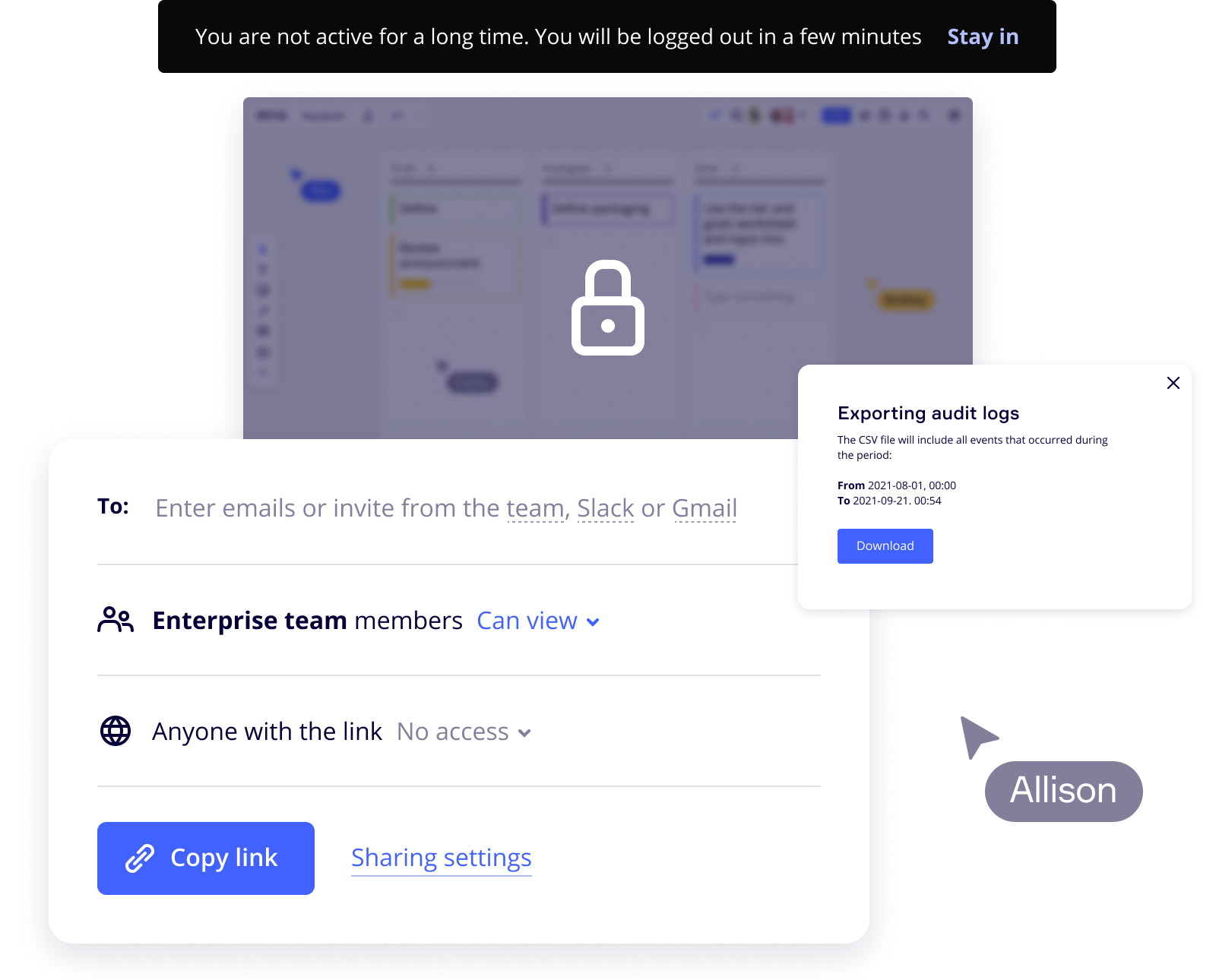The image depicts an application screen with a predominantly white background and elements in gray and black. The interface features three distinct sections. At the top, a bold black rectangle contains white text that reads, "You have not been active for a long time. You will be logged out in a few minutes. Stay in." This notification is prominently displayed, drawing immediate attention.

Beneath this notification is a grayed-out rectangle featuring a white padlock icon, indicating that the screen is locked. The padlock suggests restricted access or that certain features are not currently available.

The bottom section of the image displays a smaller, white window with text instructions. This window instructs users to "Enter emails or invites from the team, Slack, or Gmail." Below this directive, additional text indicates the level of access: "Enterprise team members can view," followed by "Anyone with the link, no access." This suggests that the app offers different levels of permission for various users, enhancing security and privacy.

The overall layout is clean and structured, using minimal color to emphasize the critical areas of interaction and notification.